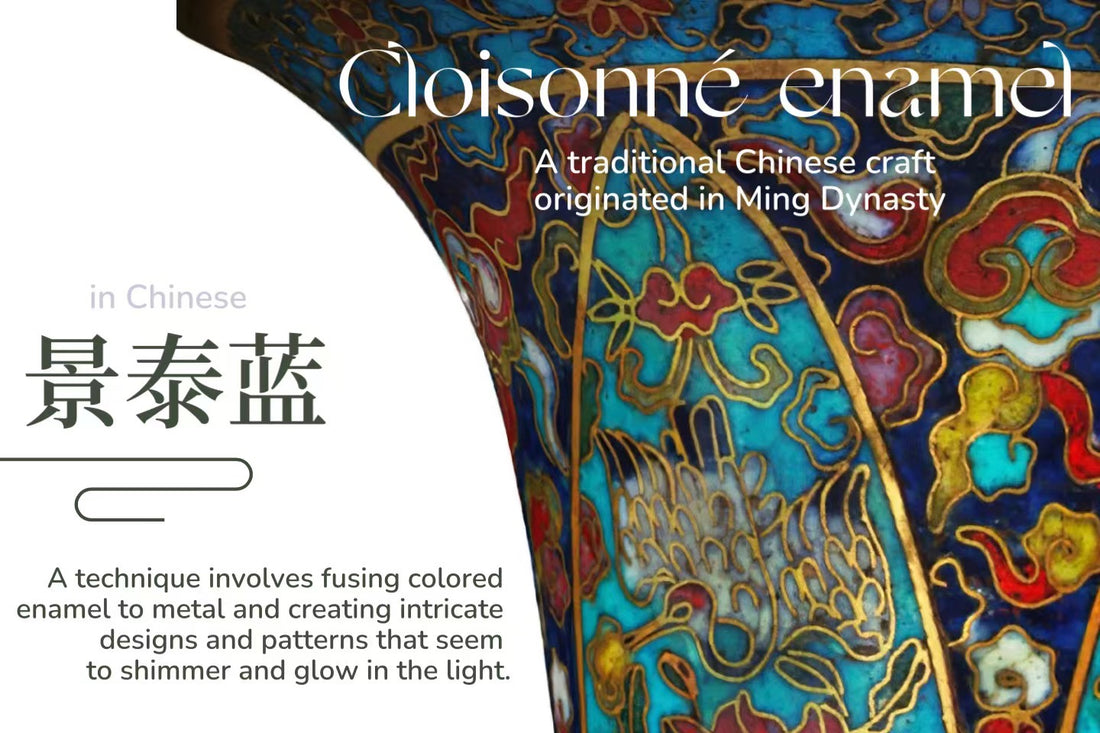This image displays an exquisite example of cloisonné, a traditional Chinese craft that originated during the Ming Dynasty. The photograph showcases a vibrant vase adorned with golden borders outlining each symbol. The intricate designs feature birds, clouds, and flowers, all meticulously crafted to create a stunning visual effect. On the left side of the image, the name of this art form is written in Chinese, accompanied by a description explaining the technique. Cloisonné involves fusing colored enamel to metal, resulting in designs and patterns that shimmer and glow in the light, highlighting the artisan's exceptional skill and attention to detail.